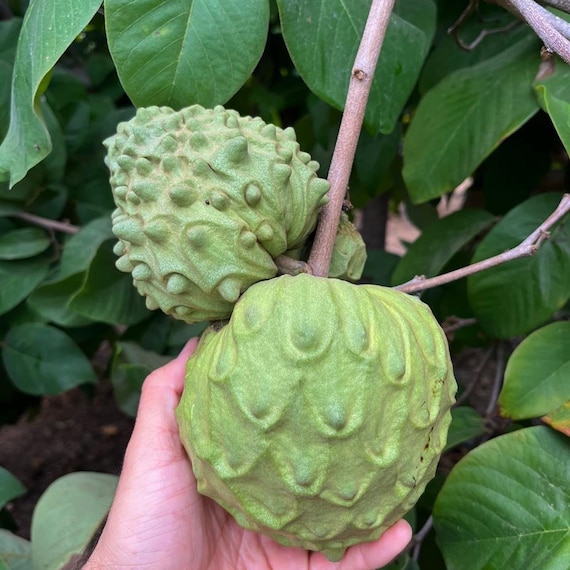The image captures a close-up view of two green round fruits known as Cherimoya, also referred to as sugar apples, hanging from a light brown stem. One of the fruits, held by a white person's left hand with the palm facing the viewer, dominates the bottom center of the photograph. This fruit is slightly bigger and more rounded, showcasing a textured, scaly surface with raised patterns of varying green shades. The second fruit appears toward the top left, slightly behind the central fruit, and is more tapered towards the bottom. Surrounding the fruits are numerous large, flat green leaves that might belong to the Cherimoya plant, with one noticeable yellowish leaf on the right side. The picture, taken in a square format, has no text or numbers and focuses on the detailed, realistic representation of the fruits, stem, and leaves, against a backdrop that includes dirt at the bottom left.